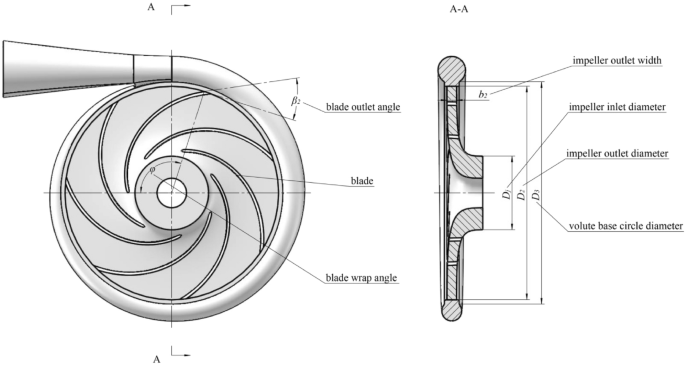This image presents a detailed, black and white diagram of a mechanical component, likely part of an impeller system. On the left side, labeled "A," there's a photograph of a cylindrical item with a conical extension, featuring multiple labeled sections: blade outlet angle, blade, and blade wrap angle. This section focuses on the intricate geometry of the blade arrangement. On the right side, labeled "AA," there's another photograph of a more oblong object with rounded ends, also with multiple labeled arrows. These labels, from top to bottom, are impeller outlet width, impeller inlet diameter, impeller outlet diameter, and volute base circular diameter, detailing the various dimensions and structural features of the impeller. Both images serve to provide a comprehensive view of the component from different angles, highlighting the critical measurements and functionalities.